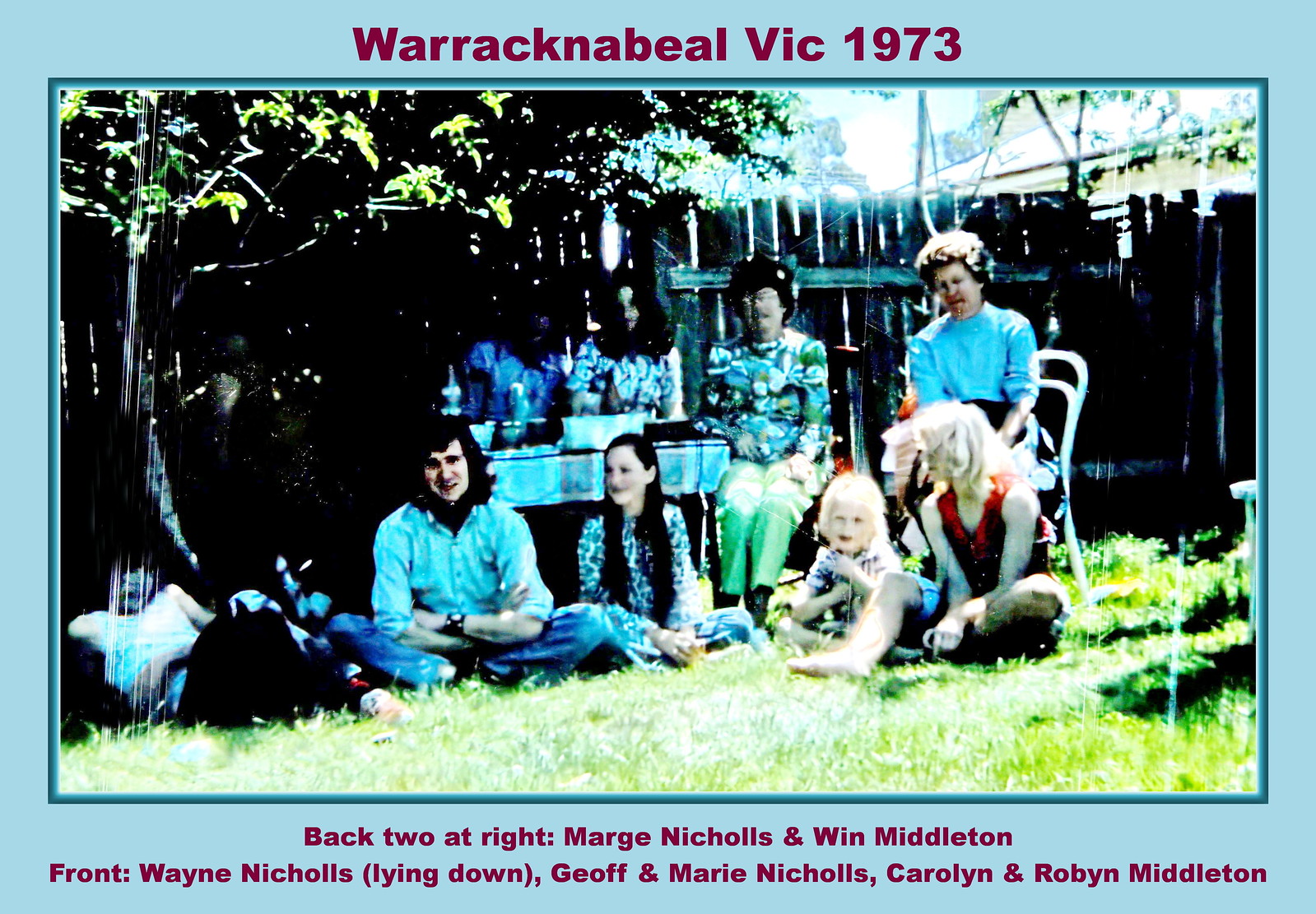The image depicts seven people outdoors, with some looking into the camera and smiling. Encased in a light blue border with red text at the top and bottom, it reads: "W-A-R-R-A-C-K-N-A-B-E-A-L, Vic, 1973" at the top, and "Back to at right, Margo Nichols and Wynne Middleton; front, Wayne Nichols (lying down), Jeff and Marie Nichols, Caroline and Robin Middleton" on the bottom. This nostalgic, sun-damaged photograph from the 1970s features high contrast and saturation, providing a glimpse into a sunny day where the group appears to be enjoying themselves in a backyard setting, possibly by a fence. Some individuals sit on the grass, while others use chairs. There's also a small table in the background, adding to the casual and friendly atmosphere of the scene.